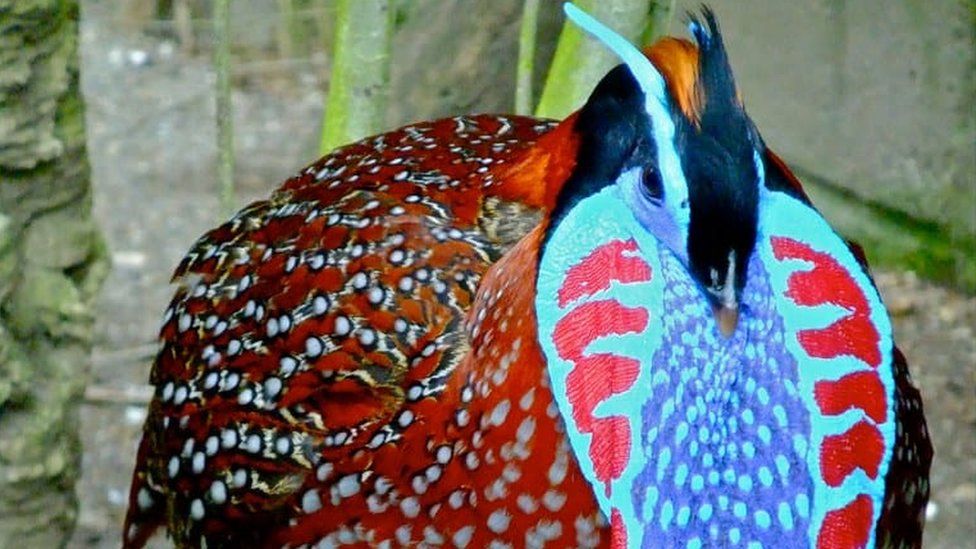This outdoor photograph captures a vibrant and striking Trigopan bird, prominently positioned in the center of the image. Rendered in mesmerizing detail, the bird flaunts a large round body cloaked in rich red feathers speckled with distinctive white spots encircled by black. Its face is oriented to the right, showcasing a black head adorned with a dramatic display of white feathers around the eyes, extending outward. Crowning its head and trailing down its neck is a fiery red plume. Adding to its colorful appearance, a striking long snood extends forward, featuring a red and white border with an intricate blue and white polka-dotted pattern.

The photo's blurred background suggests a forested environment, with indistinct trees lending a sense of depth and a natural habitat feeling. However, a concrete structure hints at the possibility of a controlled environment, such as a zoo enclosure. In the foreground, the bird's elaborate chest plumage reveals a captivating mix of blue with white polka dots, framed by red and white stripes. The overall appearance of the Trigopan is further enhanced by the vivid red, black, and orange hues that blend seamlessly with the white spotted pattern on its wings and back.

With its intricate and colorful feather patterns, the Trigopan stands out as an extraordinarily beautiful creature in this natural yet seemingly managed setting, truly embodying the artistry of nature.